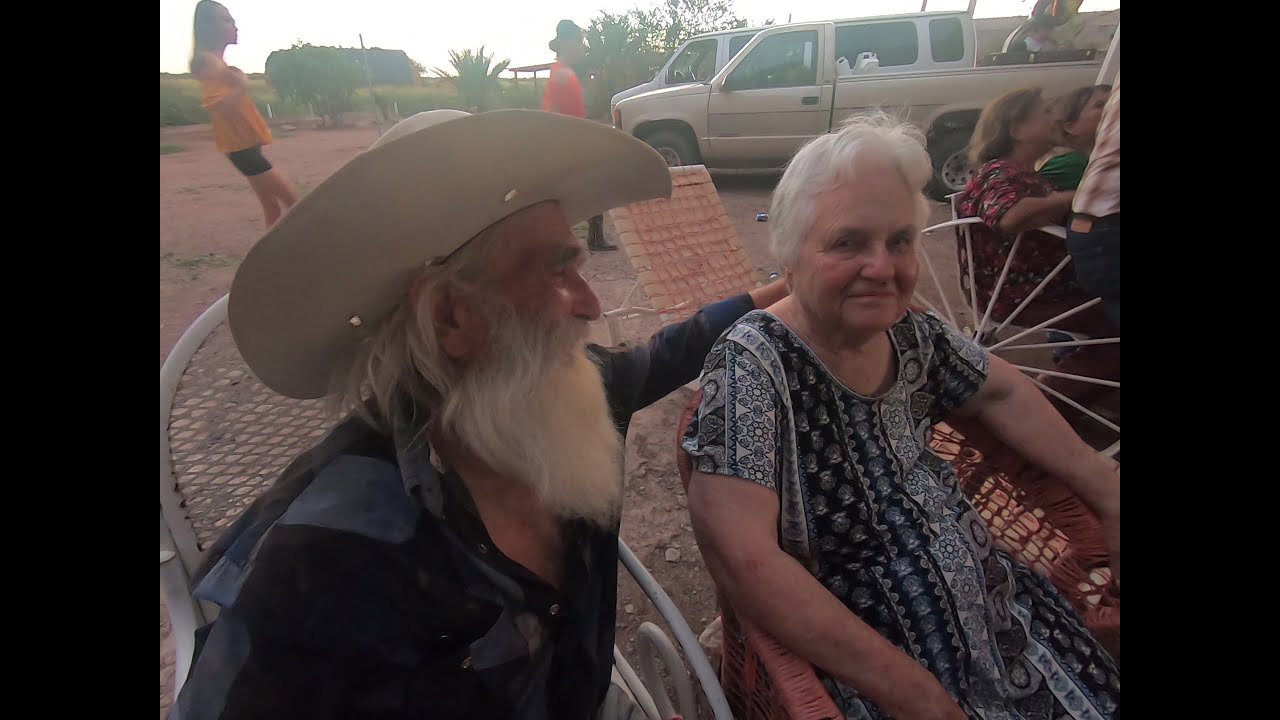In this outdoor photograph captured in an open field, the focus is on an older couple seated in the foreground. The man, distinguished by his white cowboy hat and blue shirt adorned with lighter shades of blue, has a long white beard and matching mustache. His slightly disheveled gray hair extends to his shoulders. He rests his left hand affectionately on the shoulders of the woman beside him. The woman, with short gray hair, is wearing a black and white patterned dress and sits on a red-colored, weaved chair. She faces the camera with a smile.

Behind the couple, the setting reveals a busy scene with several other people immersed in their activities, giving a communal and lively atmosphere to the image. Directly to the right of the couple, a few individuals are seated, while in the distance, younger individuals can be seen; notably, one person is in a yellow shirt with black shorts, and another in a red shirt. Cars, including a light-colored pickup truck or SUV, and a white or grayish van, are parked in the background amidst the landscape adorned with plants and trees. Despite the hazy day, the scene conveys a sense of enjoyment and relaxation among all present.